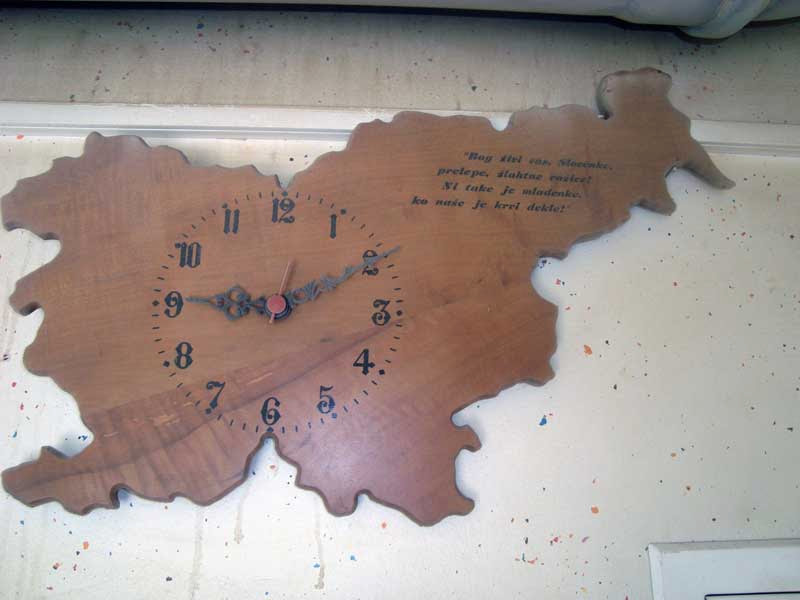This photograph features a uniquely shaped wooden clock that appears to be hand-carved, possibly into the outline of a country or an island, though the exact shape remains ambiguous. Dominating the composition, the clock is set against a white wall speckled with light dabs of blue, orange, red, and possibly gray, with some noticeable drip marks suggesting grime or spills. The wall reveals its identity as such with a white door frame visible in the bottom right corner. The clock face, with black numerals ranging from 1 to 12, indicates the time as 9:10. The minute and hour hands are ornate, black, and feature intricate scrollwork designs, while the second hand is a striking red. There is an inscription in another language, written in black script, located at the upper right part of the clock. Near the top, a raised edge or lip can be seen, and the wood itself has a light, stained, and polished finish, contributing to its distinct and handcrafted appeal.